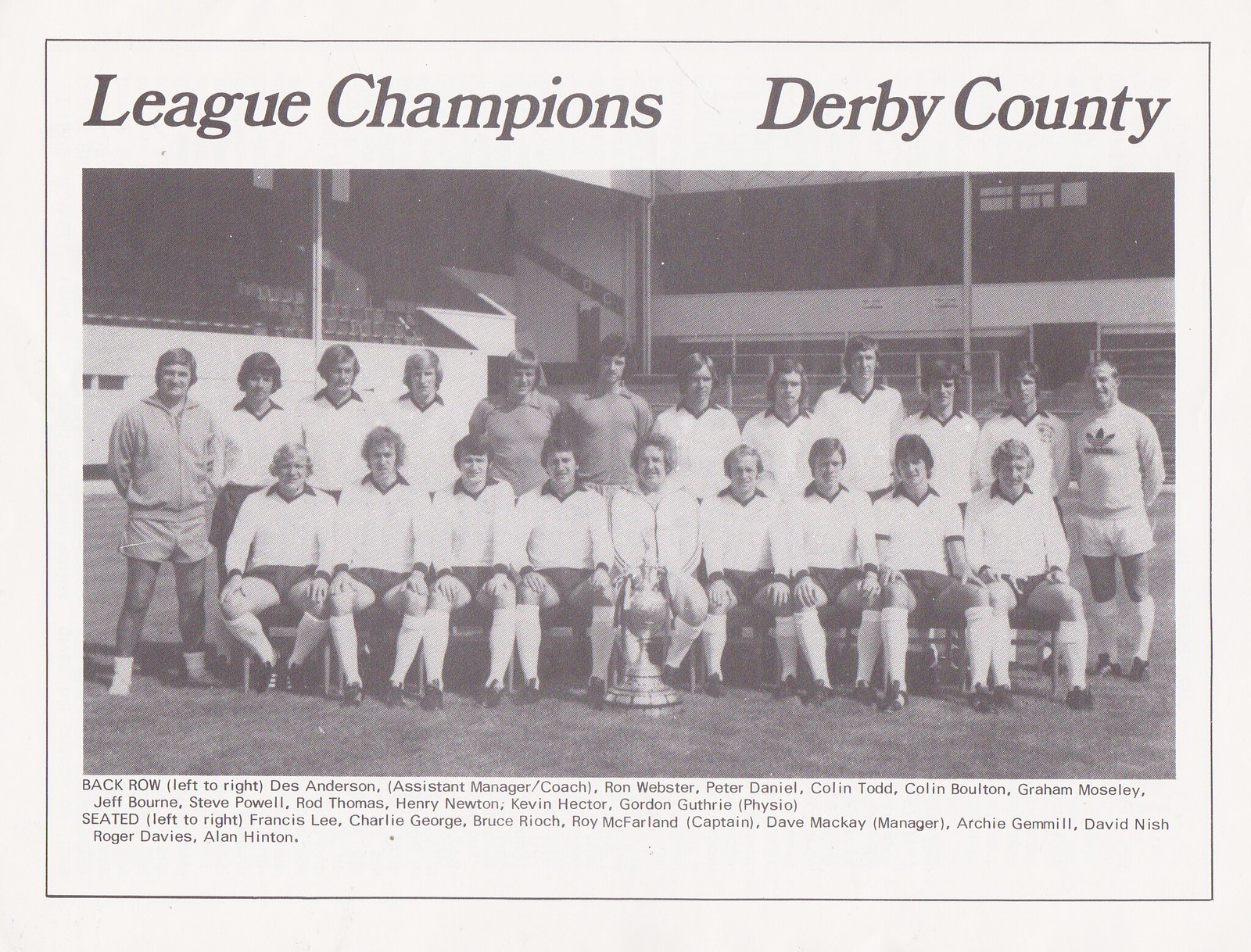The black-and-white photograph, presumably from a game day program, depicts the League Champions, Derby County, with a bold heading at the top and a thin black border around the entire page, suggesting its vintage nature. The photo features two rows of soccer players clad in white jerseys with dark shorts, joined by assistants in darker t-shirts at the back and a coach on the left in a lighter-colored jacket and matching shorts. The image is taken on a stadium field with empty seats in the background, exuding a formal atmosphere. In the front center, a trophy rests on the ground, indicating their championship status. All team members are looking directly at the camera, capturing a moment of pride. The listing below identifies each individual: 

- **Back row, left to right:** Des Anderson (assistant manager coach), Ron Webster, Peter Daniel, Colin Todd, Colin Bolton, Graham Mosley, Jeff Bourne, Steve Powell, Rod Thomas, Henry Newton, Kevin Hector, Gordon Guthrie (physio).
- **Seated, left to right:** Francis Lee, Charlie George, Bruce Riach, Roy McFarlane (captain), Dave McKay (manager), Archie Gemmel, David Nish, Roger Davies, and Alan Hinton.